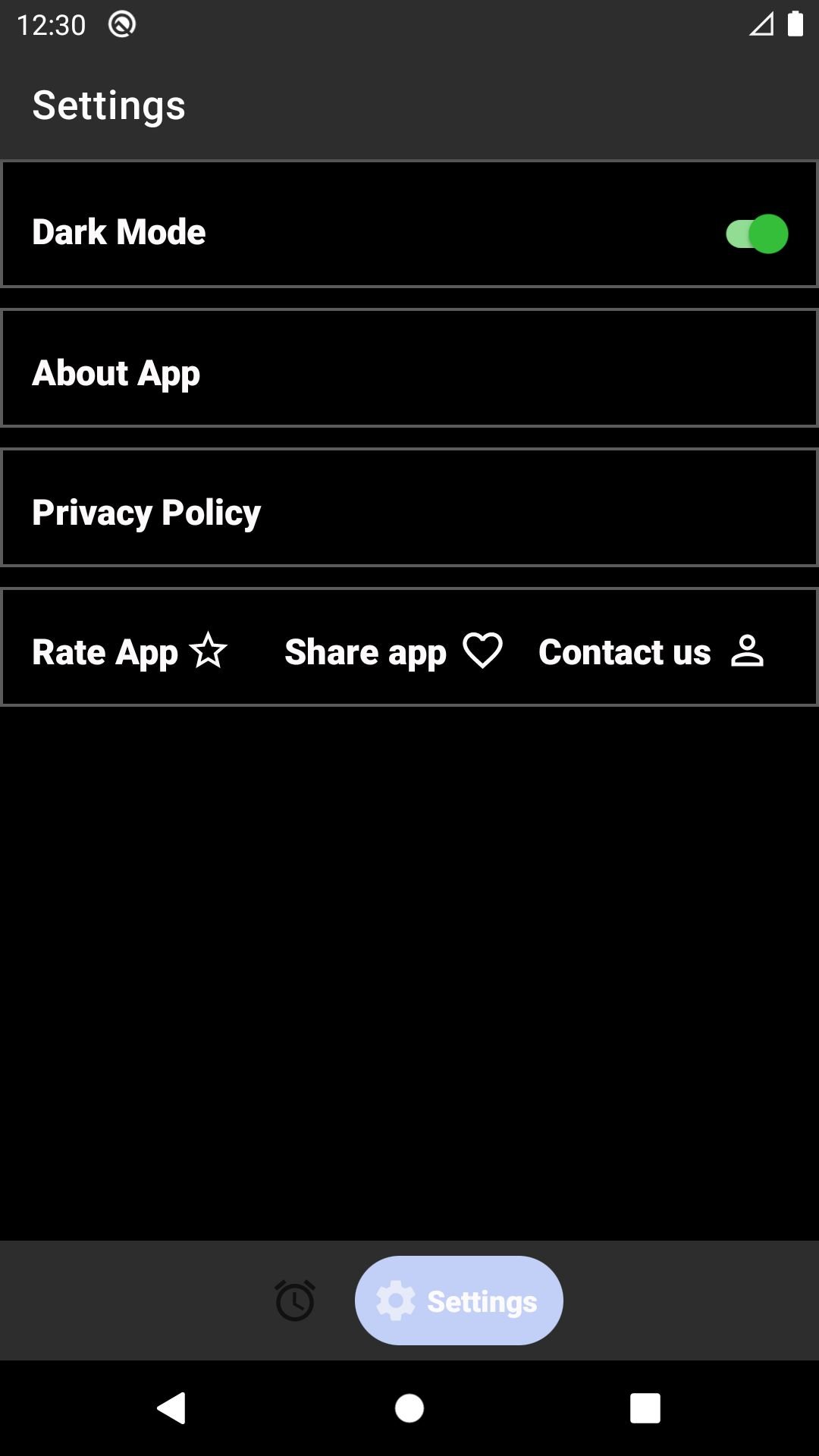The screenshot displays the settings menu of a mobile application, presented in dark mode. At the top of the screen, there is a grey header with the text "Settings". Directly beneath, a black bar with white text features a toggle switch labeled "Dark Mode" on the right side, which is activated and highlighted in green. Below this toggle, there are additional menu options listed: "About App", "Privacy Policy", and "Rate App".

At the bottom of the screen, a navigation bar is visible. The first icon from the left is a store icon labeled "Rate App". Next to it, a heart icon labeled "Share App" is positioned. To the right, an avatar icon labeled "Contact Us" is displayed.

Further down, there is a grey bar featuring a black clock icon. Adjacent to it, a light purple, pill-shaped button with a gear icon and the text "Settings" is centrally located. At the very bottom, standard navigation buttons for the phone are shown with a white back triangle on the left, a home circle button in the middle, and a recent apps square button on the right.